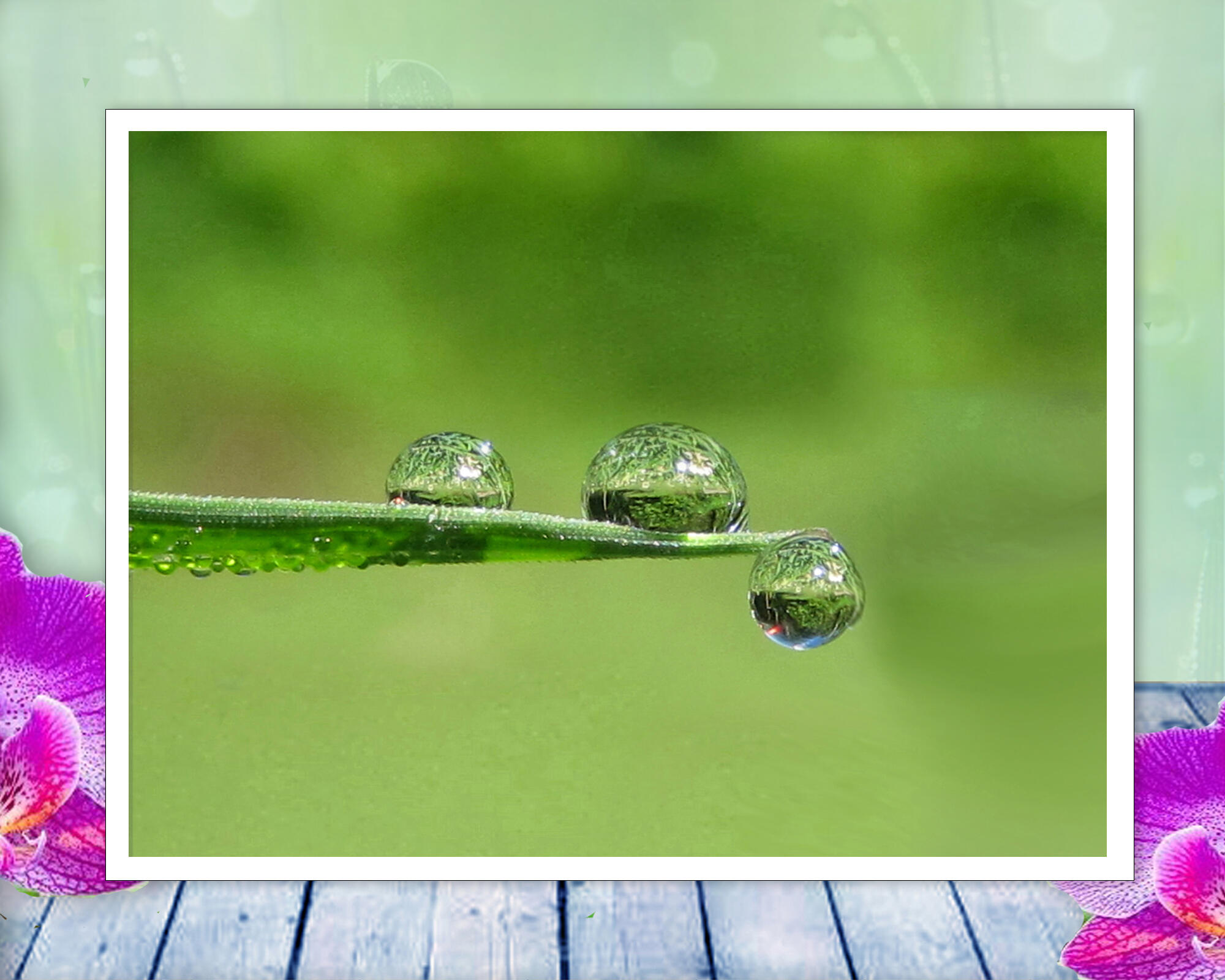The image is a composite photograph featuring a close-up of a green leaf with three spherical water droplets on its surface. The leaf extends horizontally from the left side of the foreground image, with one droplet positioned at the very tip, about to fall. The other two droplets rest on top of the leaf, reflecting intricate details of their natural surroundings. This primary photo, with its blurred green background, suggests a dewy morning setting. The foreground image is encapsulated by a thin white border and is superimposed on a secondary, slightly blurred photograph featuring a light blue wooden surface with slats. At the bottom right and left corners of this background image, large purple flowers contrast against the green and blue hues, adding a colorful frame to the serene scene of the leaf and water droplets.